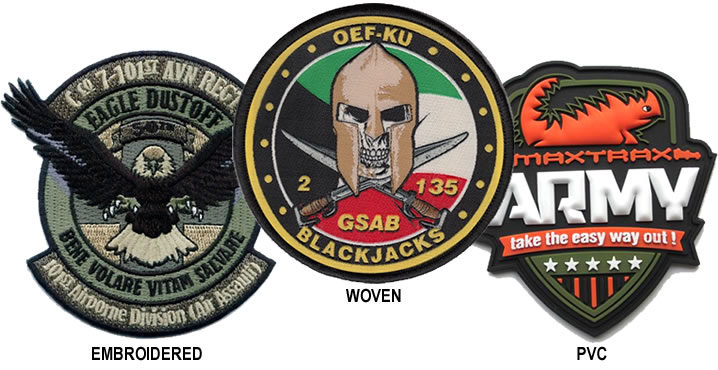The image displays three distinct military-style patches, each designed using different techniques and materials. The left patch is an embroidered design showcasing a fierce bald eagle with outstretched talons, ready to attack. It features detailed black and white feathers, with the text "CCO 7 101st AVN REGT" at the top, "Eagle Dust Off" in the middle, and additional phrases, including something in Latin and "Division Air Assassin," all embroidered in white and black threads. The center patch, created using woven techniques, depicts a skull adorned with a gold helmet and crossed swords beneath it, with the inscription "OEF-KU." The right-most patch, made from PVC, has a highly embossed appearance featuring a red dinosaur with black hair and the words "ARMY" and "Take the Easy Way Out" in raised lettering. Each patch is distinct in style—embroidered, woven, and PVC—highlighting their unique textures and visual effects.